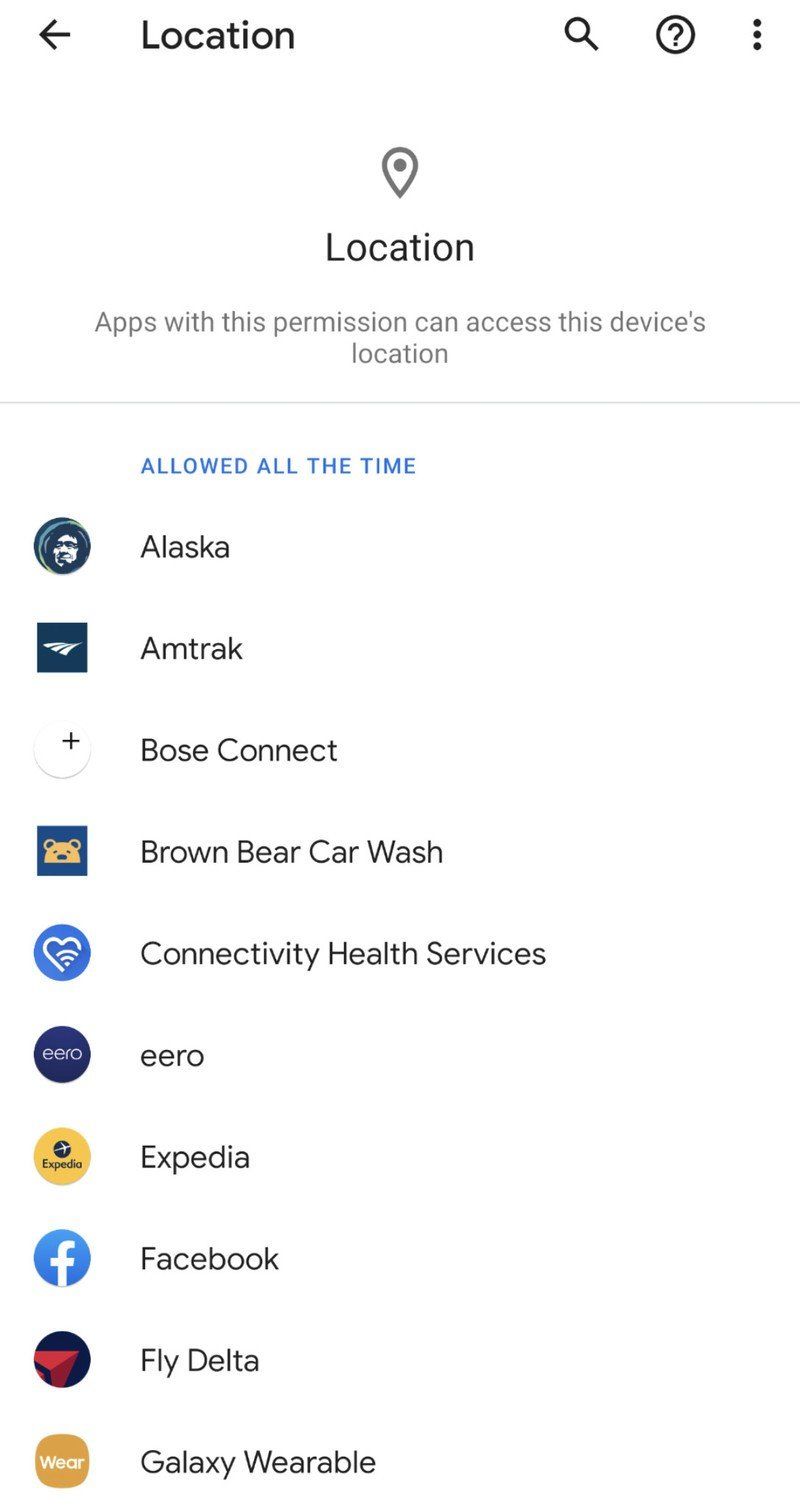The image features a clean white background at the top. Centered at the top, the heading "Location" is displayed in black text. Notably, the phrase "allowed all the time" appears in blue text, while all other text is in black. To the right corner of the top section, there are three icons: a search bar, a help icon, and a menu icon. On the top left, there is a prominent button. Below the heading, there is another instance of "Location" accompanied by a black location pin icon.

Following this, a description is provided which reads: "Apps with this permission can access this device's location." A list of apps that have location access permissions is then presented. 

The list begins with the section labeled "Allowed all the time," which includes the following apps:
1. **Alaska** - Featuring a white, navy, and green icon.
2. **Amtrak** - Displaying a navy and white icon.
3. **Bose Connect** - With a white icon and a black plus sign.
4. **Brown Bear Car Wash** - Having a blue icon with a brown bear.
5. **Connectivity Health Services** - Showing a blue icon with a white heart and Wi-Fi signal.
6. **Eero** - Represented by a navy icon and the text "Eero" in white.
7. **Expedia** - An orange icon with the word "Expedia."
8. **Facebook** - Featuring a blue icon with a white "F."
9. **Flight Data** - Displaying a navy icon with a red navigational arrow.
10. **Galaxy Wearable** - Showing a brown icon with the text "Wear" in white.